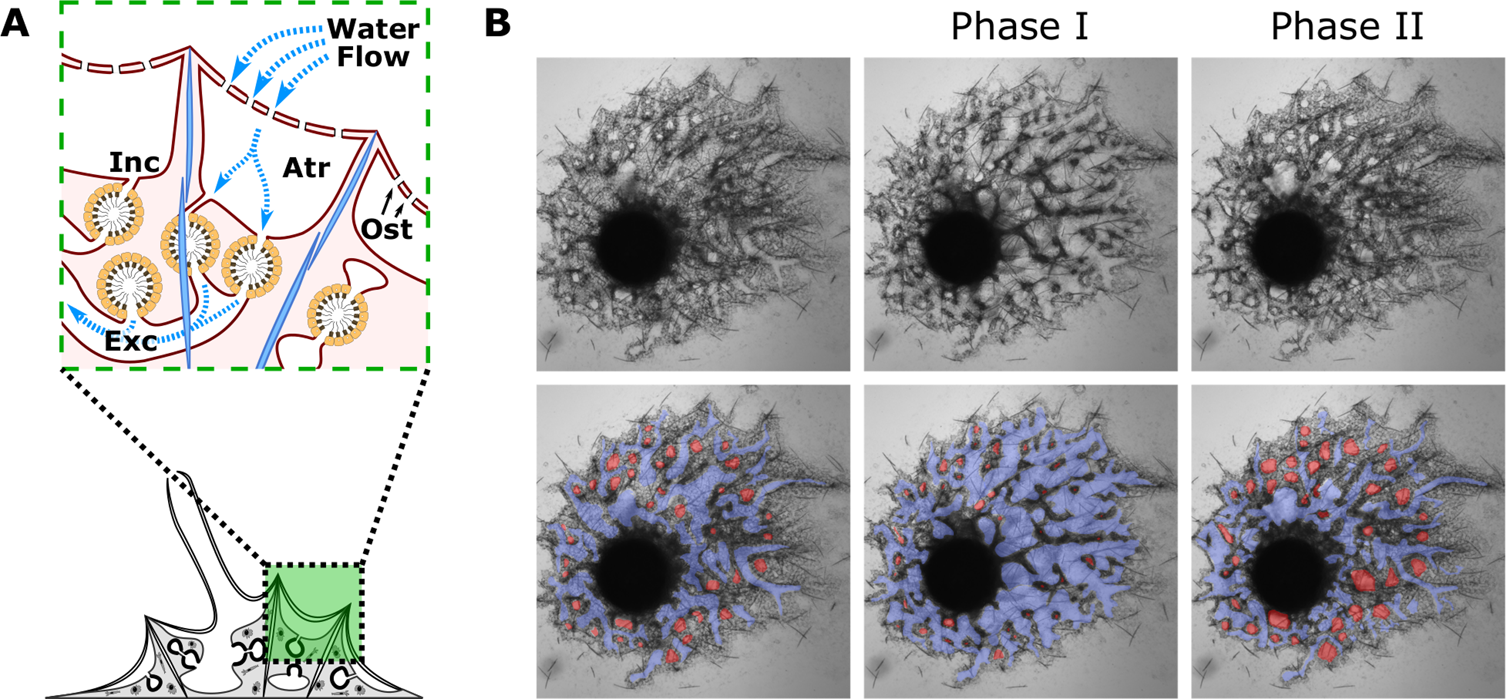The image is a detailed scientific illustration divided into two main sections, labeled A and B. Section A, on the left, contains a diagram with a green serrated-edged square. This square houses another detailed illustration labeled "water flow," highlighted by blue arrows. Key parts of the diagram are marked as INC, ATR, OST, and EXC, with orange serrated circles emphasizing significant areas. Below this illustration, it indicates magnification from a larger structure. Section B features six high-resolution microscopic images of a sample, arranged in a 2x3 grid. The top row of three images is in black and white, while the bottom row displays the sample in blue and red. The images in the second column are labeled "Phase 1," and those in the third column are labeled "Phase 2." This layout effectively showcases the progression through the phases and any changes in the sample.